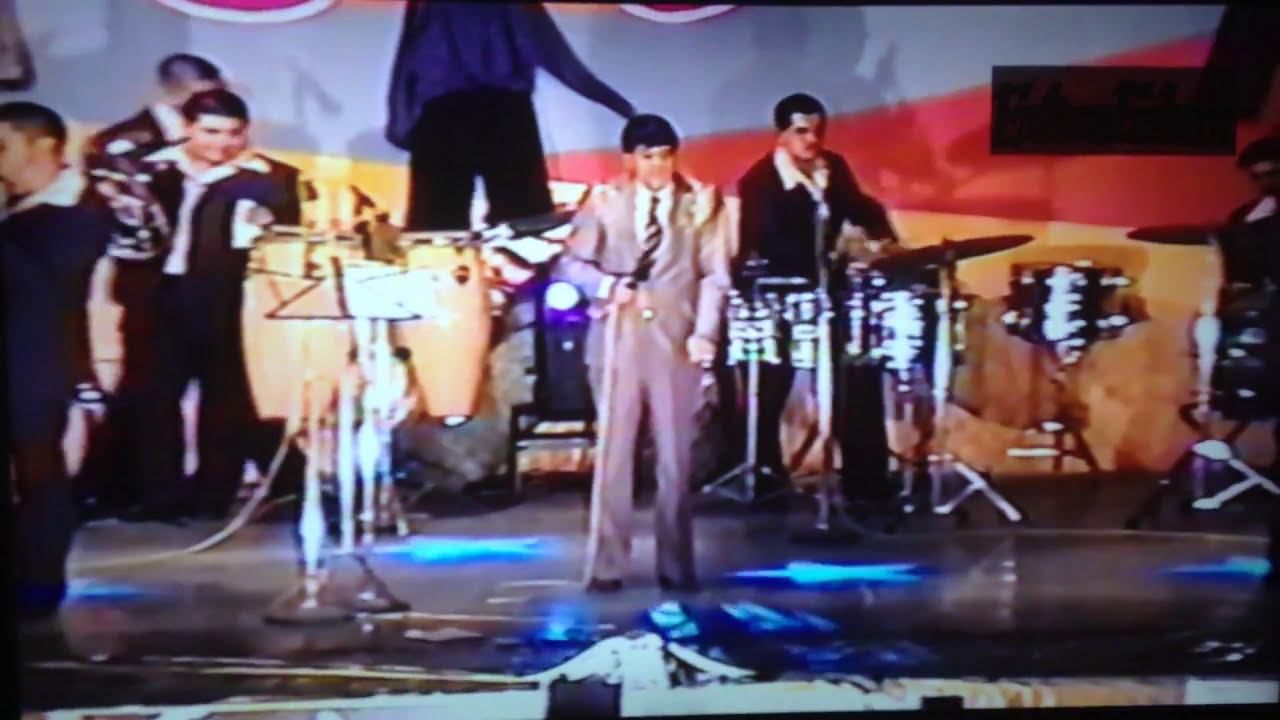The image depicts a blurry, horizontally lined rectangular stage scene, seemingly from the 1950s or 60s. Center stage, a man with short black hair dons a taupe suit and striped tie; he is holding a microphone and facing the camera. Surrounding him, several other male performers—also with short dark hair—are dressed in dark suits with white collared shirts. Notably, behind the central figure, a drummer in a black suit with a white shirt is positioned with a set of three drums and a cymbal. To the left, another instrumentalist holds what appears to be a French horn. The stage floor is silver, adorned with blue stars, while the background is characterized by a banner or wall featuring large red and gray stripes. High in the background, another individual, mostly obscured, appears to be wearing a blue top and black pants. The image captures a dynamic band performance but lacks clarity, making it difficult to discern all details precisely.